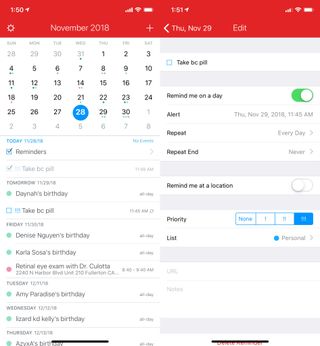This image features a November 2018 calendar with a red border at the top. The top left corner displays the number "150," and the top right corner shows icons for cellular connection, wireless signal, and a full battery. To the left, a gear icon is followed by the text "November 2018." The calendar spans from the 1st to the 30th of November, with the 28th particularly highlighted by a blue circle. 

Although much of the text in the image is blurry and difficult to decipher, a checkbox labeled "Reminders" is visible and marked with a check. Next to the checkbox, text that appears to say "11-29" is partially readable, followed by "Dana's Birthday." Further down, legible text includes "Denise Nguyen's birthday," "retinal eye exam with Dr. Kolata," "Amy Paradise's birthday" on a Tuesday, and "Lizard Kid Kelly's birthday" on a Wednesday.

On the right side of the calendar, "November 29" is prominently displayed at the top, beneath which there is an unchecked box labeled "take BC pill." Below this, the phrase "Remind me on a day" appears, with the option highlighted in green.